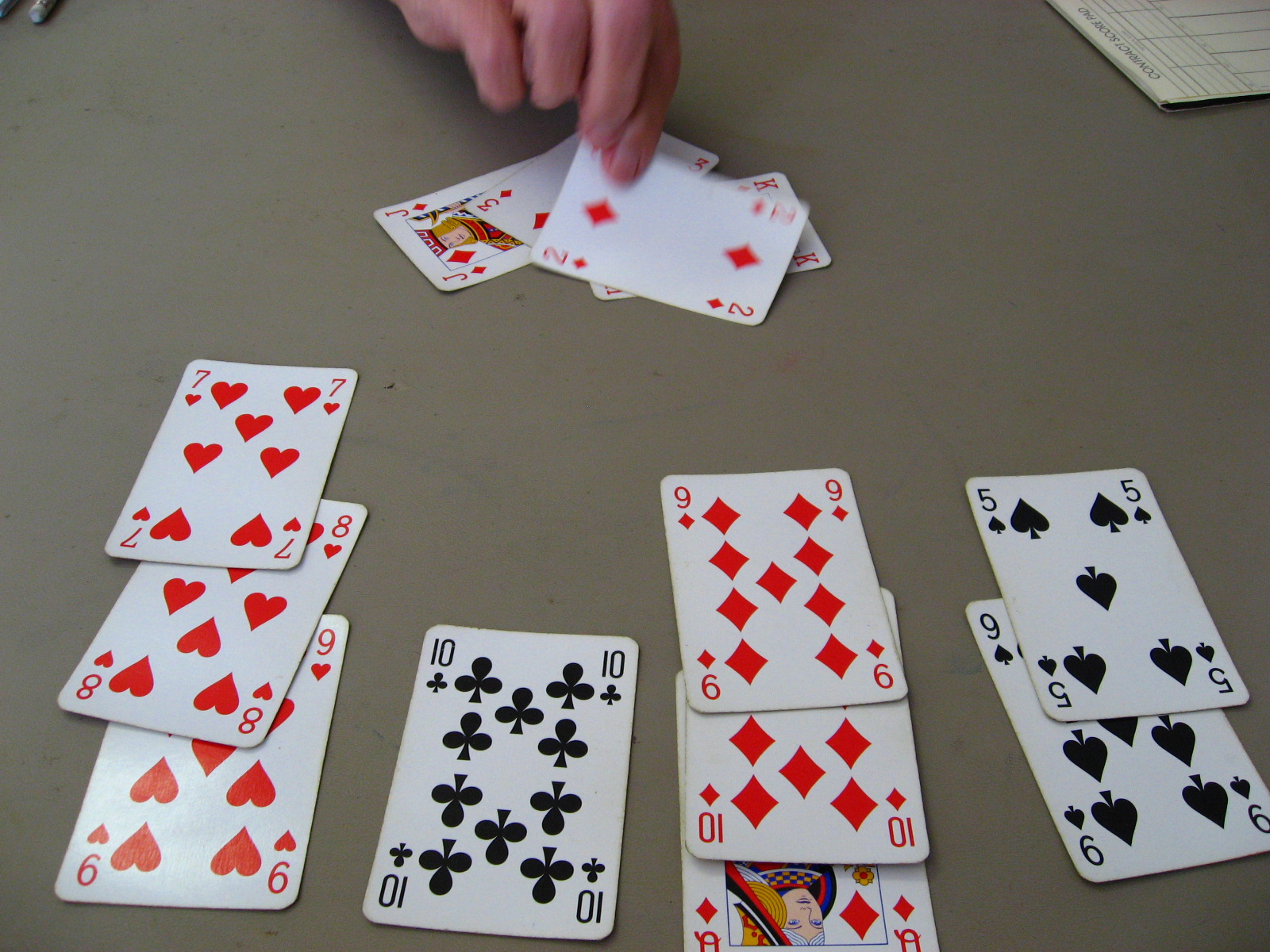This image features an assortment of playing cards meticulously arranged in four columns. Starting from the left, the first column displays a descending sequence of hearts, including the Nine of Hearts at the bottom, followed by the Eight of Hearts and the Seven of Hearts on top, all in vivid red. The second column showcases a lone black Ten of Spades. The third column contains three red diamond cards, starting with the Queen of Diamonds, followed by the Ten of Diamonds, and the Nine of Diamonds. The fourth column presents two black spade cards: the Nine of Spades at the bottom and the Five of Spades above it.

In the background, there's a scattered pile of playing cards. Among them, we can distinctly identify a Jack of Diamonds, the Joker, and a Three of Spades. Additionally, a King card appears slightly obscured, revealing only its red-colored details without showing the suit. A Two of Diamonds is partially visible, being held at its corners by a hand, of which only the fingertips are seen in the frame, gently pinching the card together.

The detailed arrangement of the cards, coupled with the various colors and suits, create a visually engaging and intricate display.